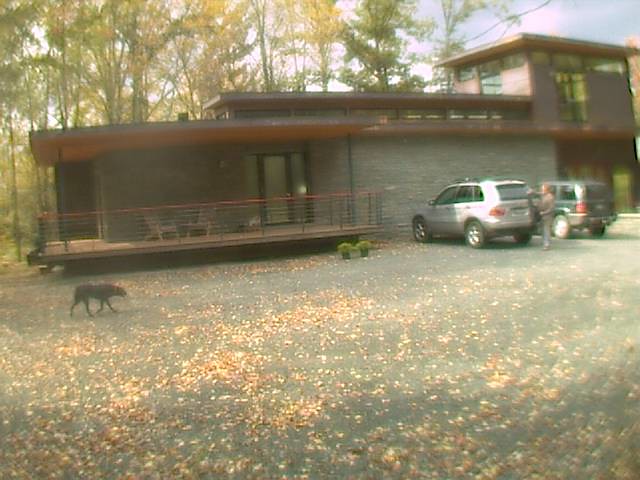On a sunny autumn day, a blurry photograph captures a modern, right-angled house exuding contemporary architectural design. In the foreground, an animal strolls past two parked SUVs, with a man reaching up towards the back of one vehicle. The house features a patio enclosed by a railing, furnished with two chairs, and flanked by two potted plants. Behind the structure, a mix of trees with vibrant yellow and green leaves creates a picturesque backdrop. A large expanse of pavement, scattered with brown fallen leaves, lies in front of the house, encapsulating the essence of a crisp fall day.